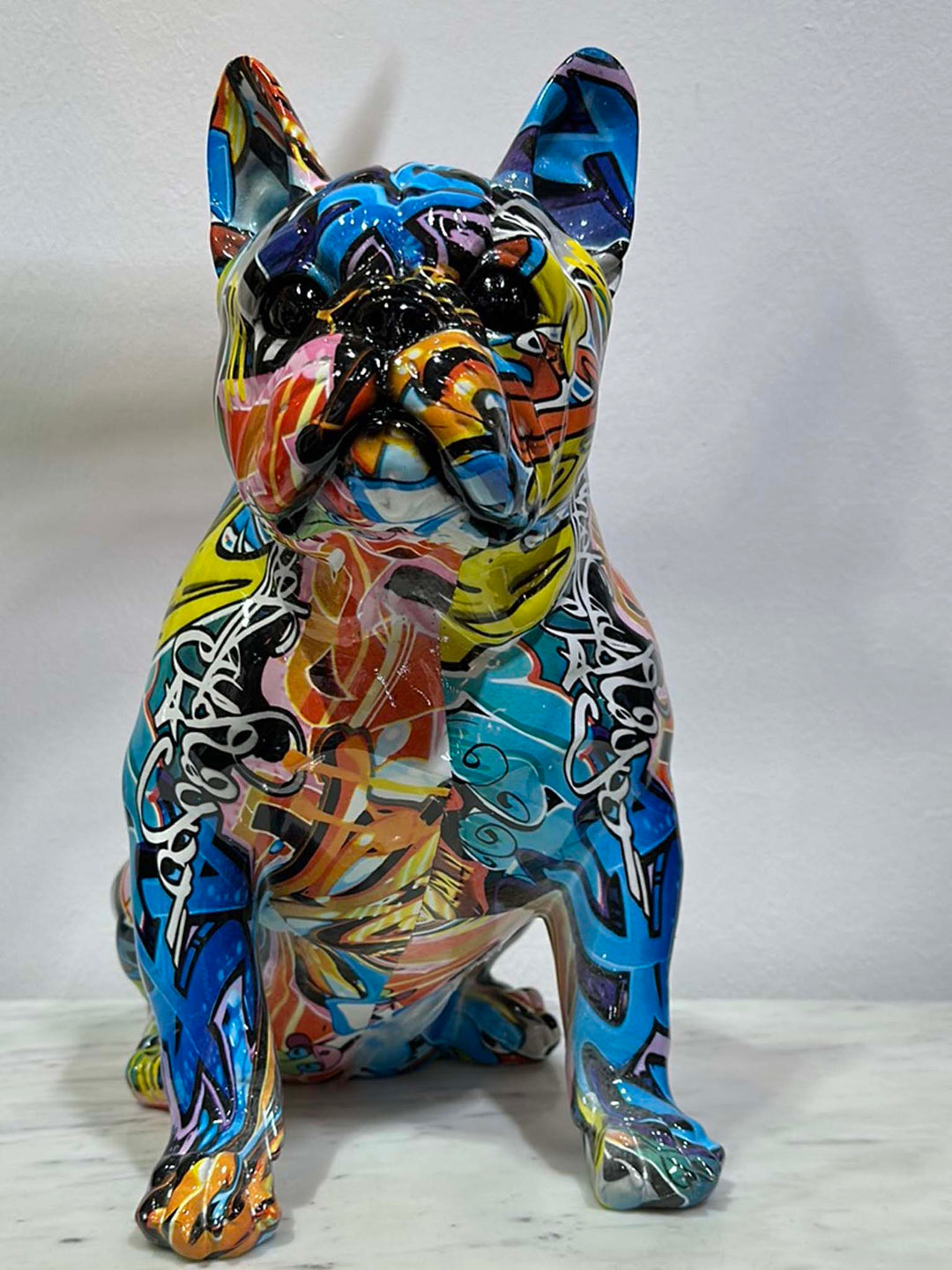This image features a striking figurine of a French bulldog, crafted likely from a shiny, glazed ceramic material. The dog is sitting, facing the camera, with its ears perked up and solid black eyes that seemingly peer directly at the viewer. Its nose and mouth are also outlined in black, providing a stark contrast to the vibrant, swirling graffiti-like patterns that envelop the entire figurine. The body showcases an array of colors, including red, black, yellow, several shades of blue, light purple, green, and pops of orange, creating a visually arresting mosaic of patterns and styles. Notably, white script-like text elegantly scrolls down its shoulders and front legs, though the exact words are indiscernible. The bulldog sits on a white and black surface, with a deliberately placed background, possibly a paper, suggesting that the photo could be intended for a catalog, gallery, or an artist's portfolio. The overall effect is a mesmerizing confluence of color and design, reminiscent of the best street art transposed onto a three-dimensional canine canvas.